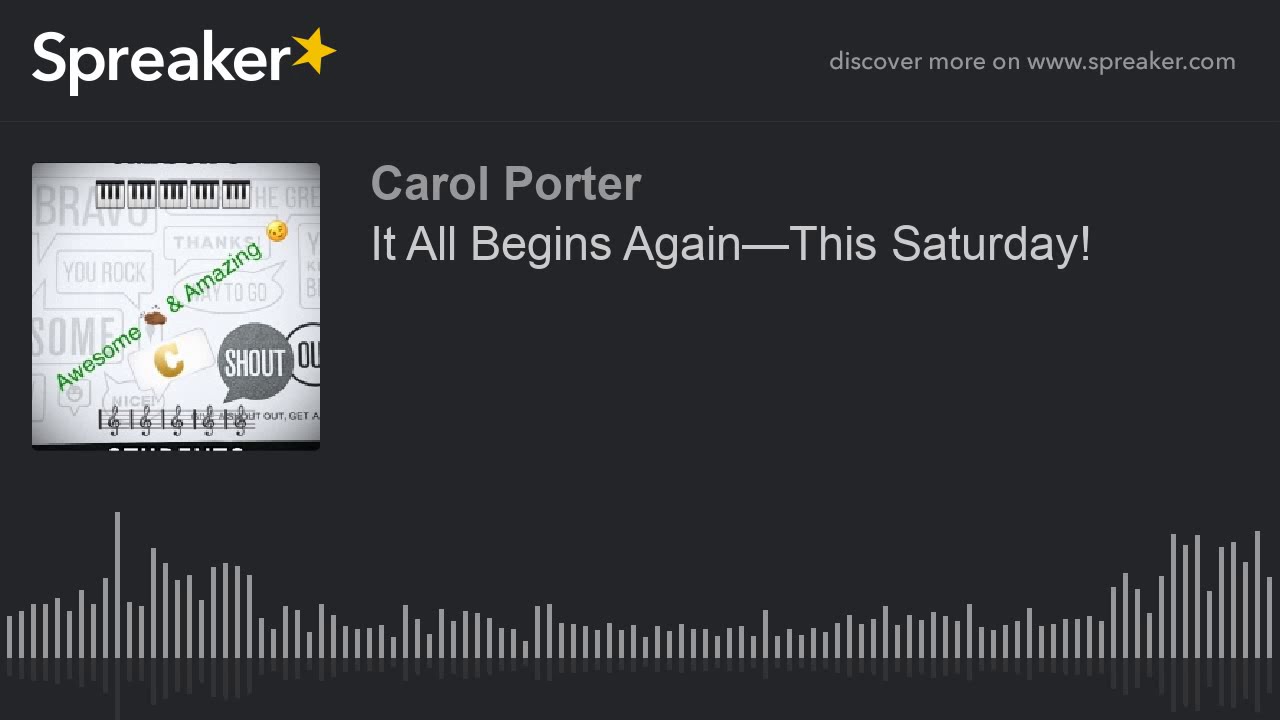The image appears to be an advertisement for a podcast on the Spreaker platform, depicted on a horizontal, black background. In the upper left-hand corner, "Spreaker" is prominently displayed in white sans-serif letters with a yellow star of uneven sides positioned at the end of the word. In the upper right-hand corner, the words "discover more on www.spreaker.com" are written in small, gray font. Below "Spreaker," there is a colorful square image showing piano keys and musical notes, overlaid diagonally with the words "Awesome and Amazing" in green font. Emerging from the notes, a gray speech bubble contains the word "shout." To the right of this square, the name "Carol Porter" appears in gray font, followed by the text "It all begins again this Saturday." Finally, spanning the bottom of the image are multiple gray vertical lines of varying lengths, resembling sound waves or equalizer bars.